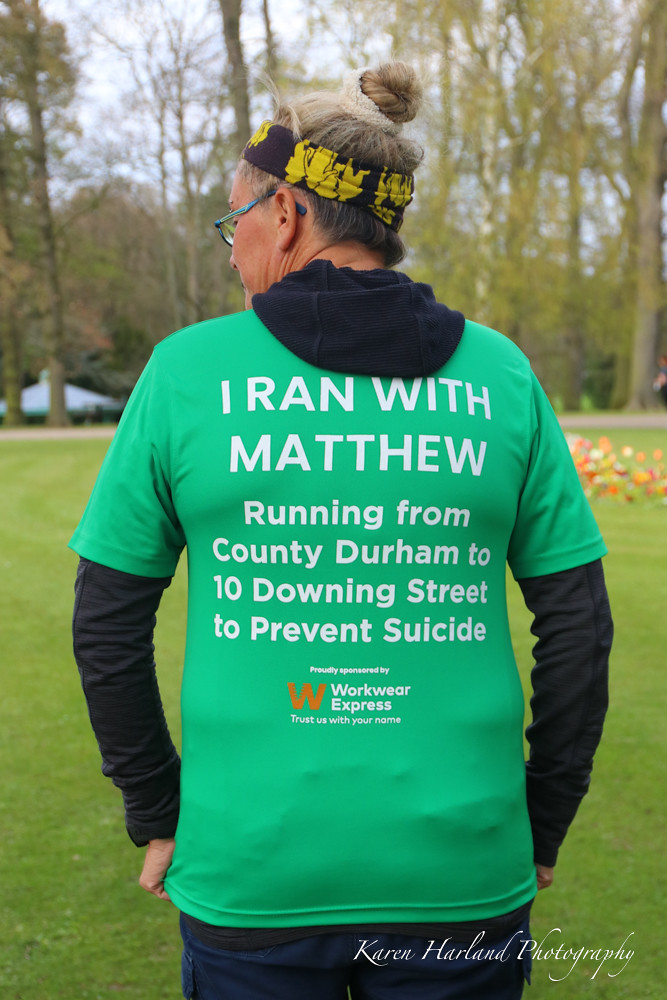This rectangular photograph captures a close-up view of a middle-aged woman standing outdoors in what appears to be a large grassy park. She's facing away from the camera, standing amidst a spread of flowers with a tree line visible in the distance. On the left side of the image, partially obscured by trees, there is a building structure. The woman is dressed casually in jeans and a long-sleeved black hoodie. Over the hoodie, she wears a distinctive green t-shirt with white writing that reads: "I ran with Matthew running from County Durham to 10 Downing Street to prevent suicide." Below this, the shirt is emblazoned with the sponsorship details: "Proudly sponsored by Workwear Express. Trust us with your name." Adding more detail to her appearance, her hair is tied back in a bun, and she's adorned with a red and black headband and a pair of glasses. The photo is credited to Karen Harland Photography, as indicated by the text at the bottom of the image.